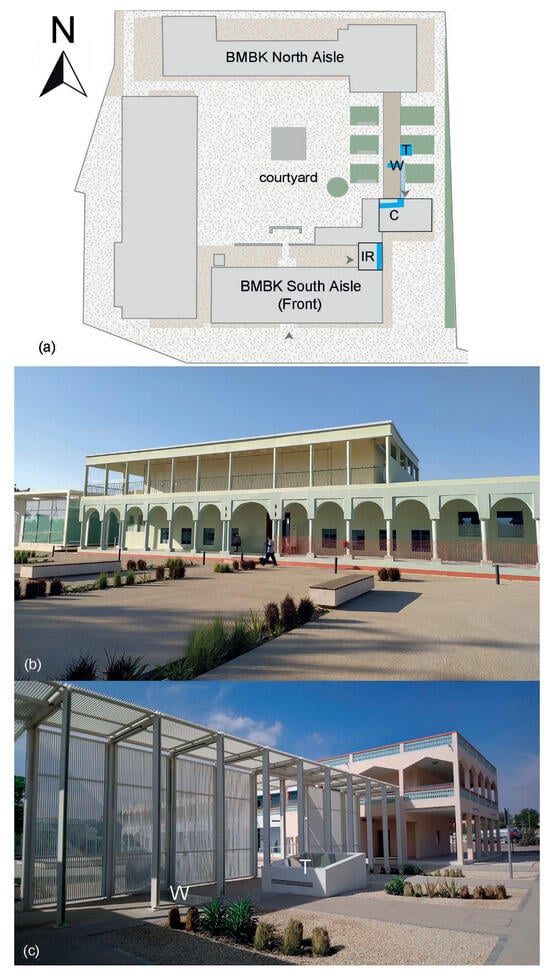The image is divided into two main sections. The top 30-40% features a detailed map of a building complex with a central courtyard labeled "Courtyard." Surrounding the courtyard are four buildings. The top building is marked "BMBK North Aisle," the bottom building is labeled "BMBK South Aisle Front," there is an unlabeled rectangular structure on the left, and a series of green bars, possibly indicating another building or a landscape feature, on the right. There is also a letter "N" with an arrow near the top-left corner, indicating the direction.

Below the map, two horizontal rectangular photographs depict the architectural details of the same buildings shown in the map. The left photograph, labeled "B," shows a modernist two-story building with porticoed walks on both floors. The ground floor features archways lined with columns, while the top floor includes a colonnade. A landscaped plaza with rows of manicured bushes and two long benches lies in front of the building. The right photograph, labeled "C," illustrates a similar building connected by a shaded walkway, likely covered with wire mesh walls and a roof. This building also features a colonnade and a top-floor porch, set against a foreground of shrubbery and paved areas.